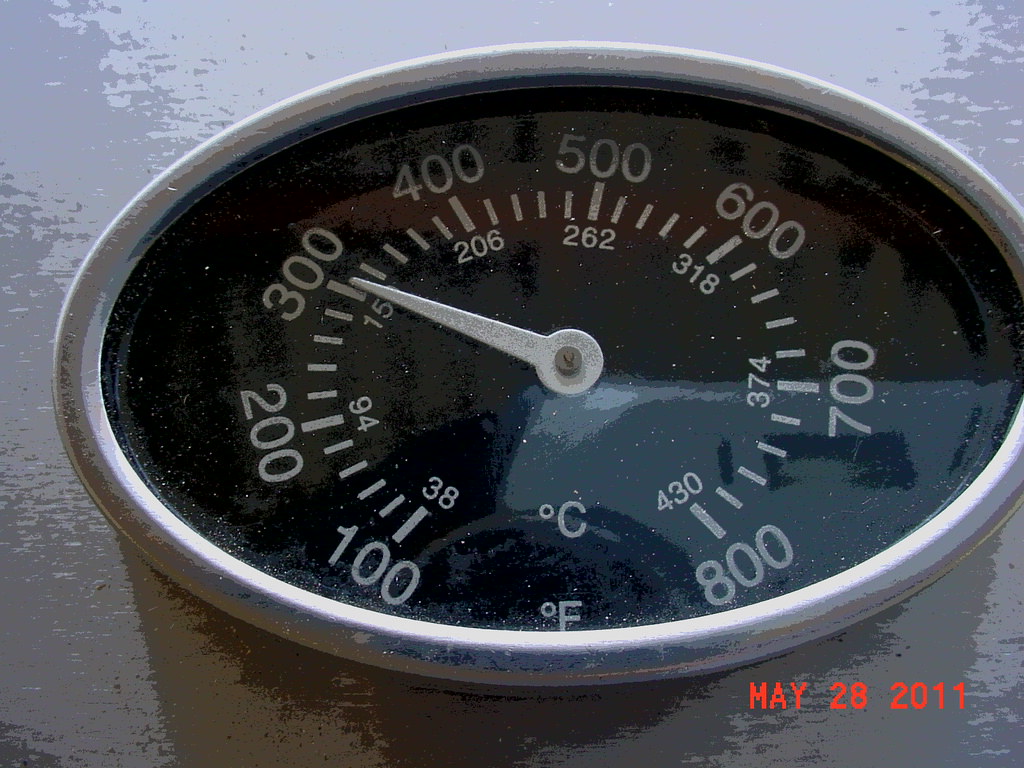A detailed black-and-white image captures the close-up of a thermostat on an outdoor barbecue grill. The photograph, with a grayscale aesthetic, highlights the intricate details of the thermostat prominently placed at the center. The device features both Fahrenheit and Celsius measurements. The Fahrenheit scale arcs from 100 to 800 degrees, marked in increments of 100, while the Celsius scale is indicated inside, ranging from 38 to 430 degrees. The face of the thermostat is black, contrasting sharply with the silver numerals and the central hand. A small screw secures the hand in the middle of the thermostat. A timestamp in red, situated at the bottom right corner, reads "May 28, 2011," providing context to the image. The focused composition and monochromatic scheme bring attention to the meticulous design and functionality of the thermostat on the grill.